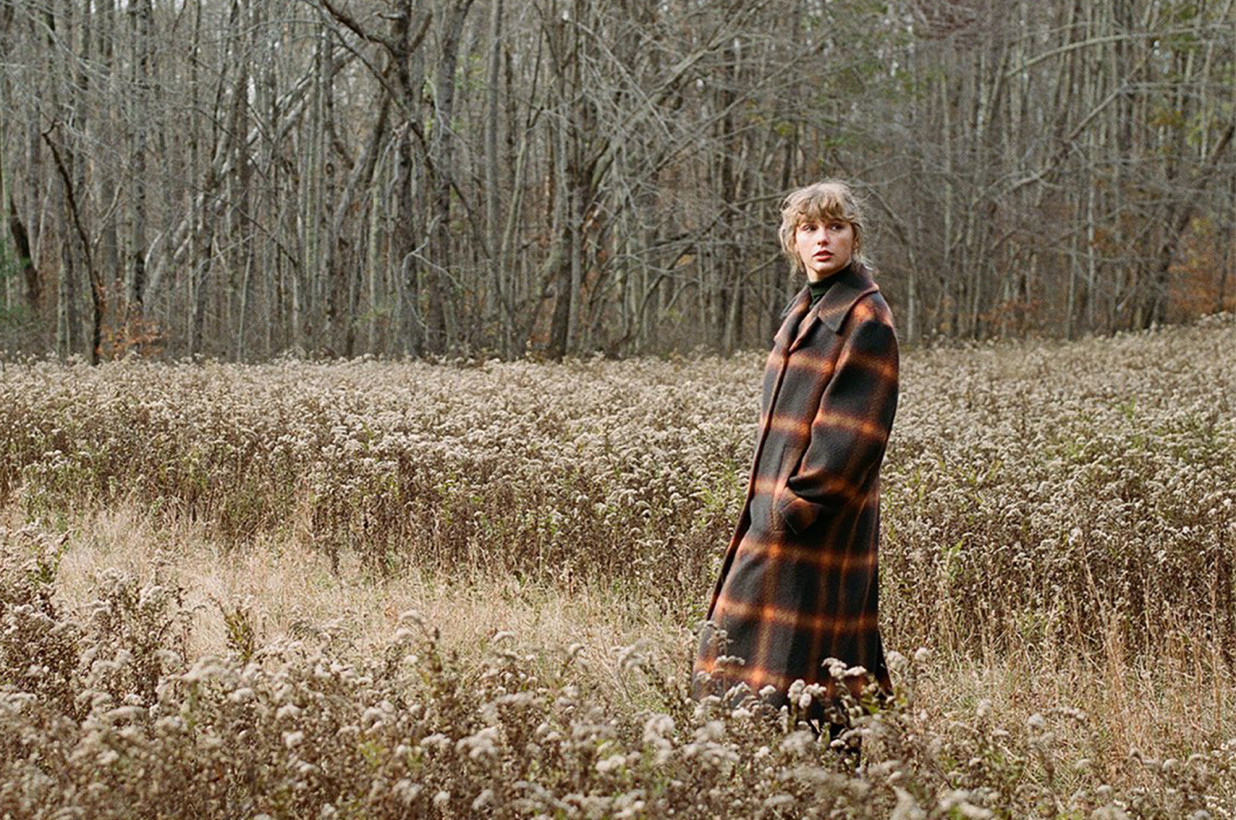In this winter scene, a tall woman reminiscent of Taylor Swift stands in a field of tall, dry, brown grasses and faded flowers, their tops dusted with white. The backdrop features sparse, skinny tree trunks, stripped of their foliage, evoking a cold, gloomy atmosphere. The woman, with her frizzy blonde hair and clear skin, is dressed in a long, dark brown or black Czech coat with orange stripes forming a grid pattern. Beneath this coat, she wears a dark turtleneck. With her hands tucked into her pockets, she gazes to her left, adding to the serene and contemplative mood of the image. The image captures a distinct winter vibe, emphasizing the dry, dormant state of the surrounding nature.